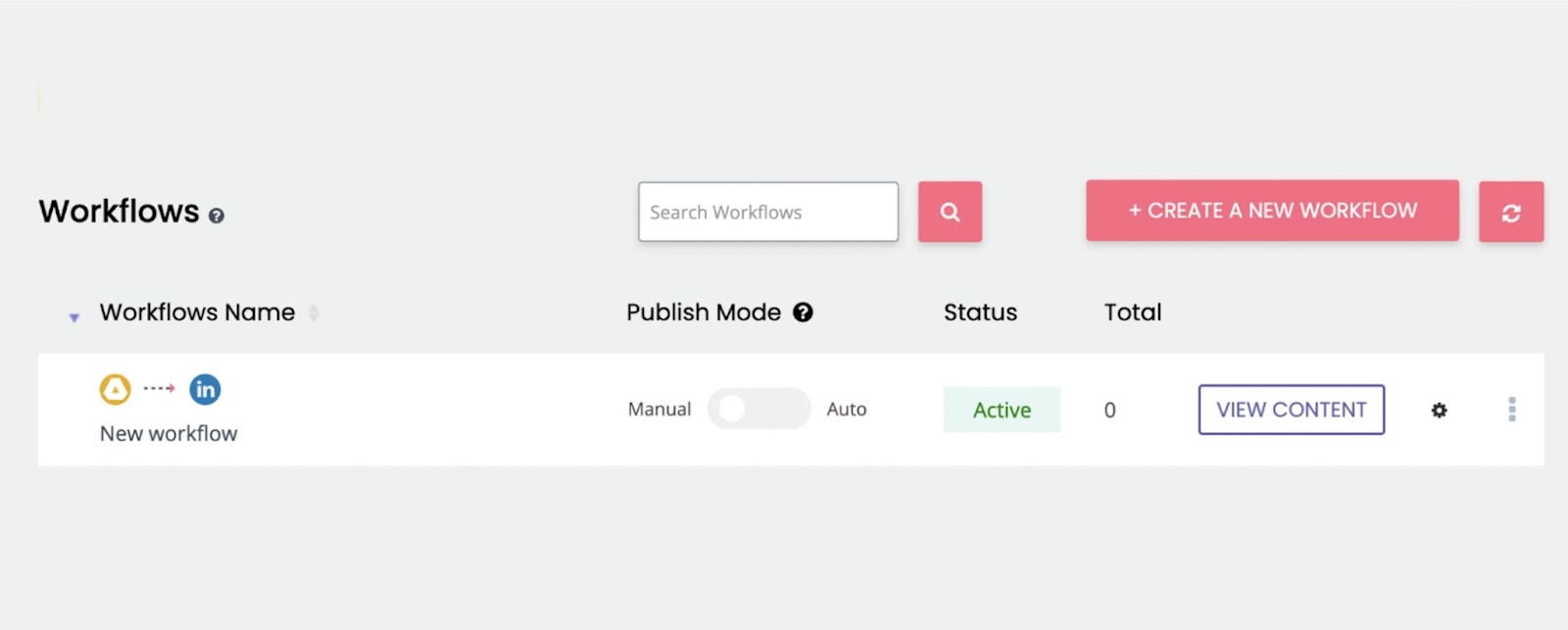This image depicts a webpage interface with a predominantly gray background. Centrally positioned towards the left, the word "Workflows" is prominently displayed alongside a small question mark icon. Below this header, the label "Workflow name" appears, followed by a long white input field spanning nearly the entire width of the image. Within this input field, there is a recycling symbol adjacent to an arrow that points towards the word "New Workflow," enclosed in a blue circle.

Further down, there is a slider toggle with options for "Manual" and "Auto," currently set to "Manual." The workflow's status is labeled as "Active" in green text. The "Total" count is marked as "Zero," and situated nearby is a purple button labeled "View Content." At the far right of this section, there is a gear icon.

Above the central section, at the top left, there's a white button labeled "Search Workflows," accompanied by a pink magnifying glass icon. To its right, a pink button says "Create a New Workflow," featuring an exchange arrow symbol.